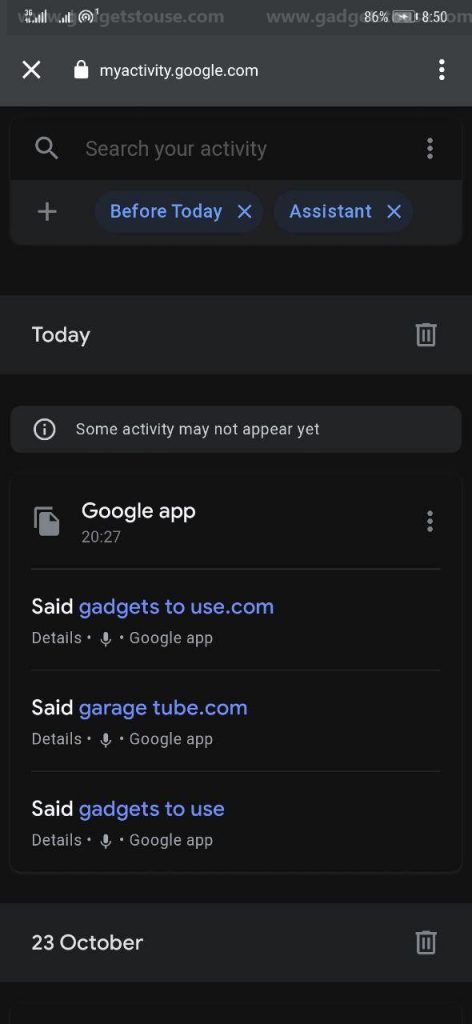Screenshot from a mobile device displaying several details: At the top, various status icons are visible, including a Wi-Fi signal, the current time of 8:50, and an 86% battery level. A watermark appears at the top, which seems to read "GadgetsToUse.com". The background of the screenshot is gray with white text, indicating the webpage is "myactivity.google.com". 

Below this section, the interface shifts to mostly black backgrounds, featuring a search bar for users to look through their activity and category filters below it, such as "Before Today" and "Assistant," which can be removed or added. Further down, under the header "Today," there's a note stating, "Some activity may not appear yet."

Specific activity logs are listed:
- "Google app, time 20:27"
- "Said gadgets to use.com"
- "Said garage tube.com"
- "Said gadgets to use"